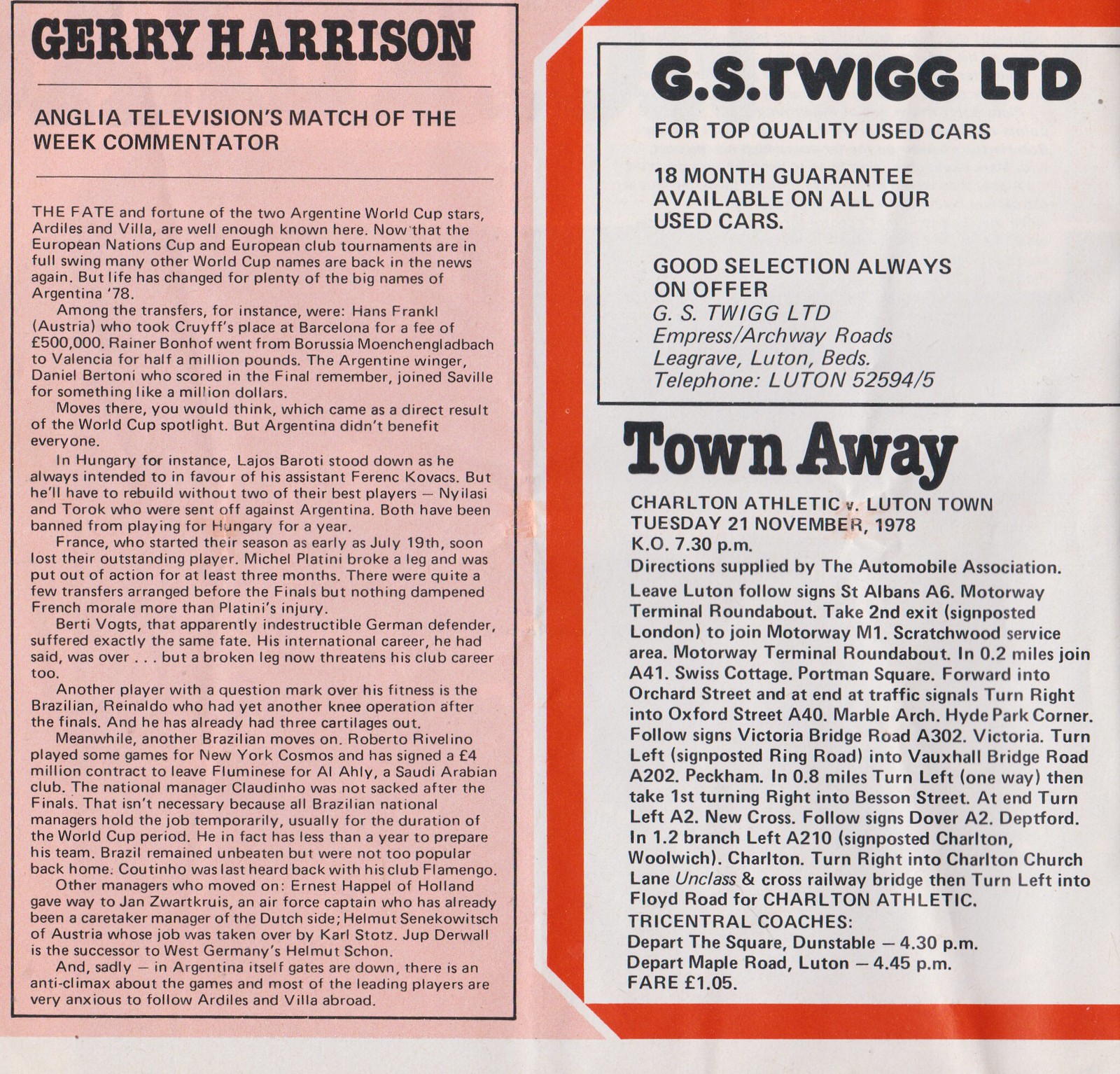The image depicts a vintage page from an old soccer magazine, likely a European football magazine, divided into two distinct sections. The left section features an article with a pink background and black text, authored by Jerry Harrison, who is noted as Anglia Television's Match of the Week commentator. The article delves into the relevance of Argentinian World Cup stars like Audley and Villa, set against the backdrop of ongoing European Nations Cup and European Club tournaments.

On the right side of the page, there are two sections with a white background and black text, each bordered in red. The top section is an advertisement for GS Twig Limited, promoting its top-quality used cars with an 18-month guarantee and a constantly superb selection, available at their location on Empress/Archway Roads, Luton. The bottom right section details an upcoming soccer match, Charlton Athletic versus Luton Town, scheduled for Tuesday, 21 November 1978, with a kickoff at 7:30 PM, including information about attending the game and associated costs.

Overall, the page captures both the spirit of football journalism and quintessential vintage advertising from the era.